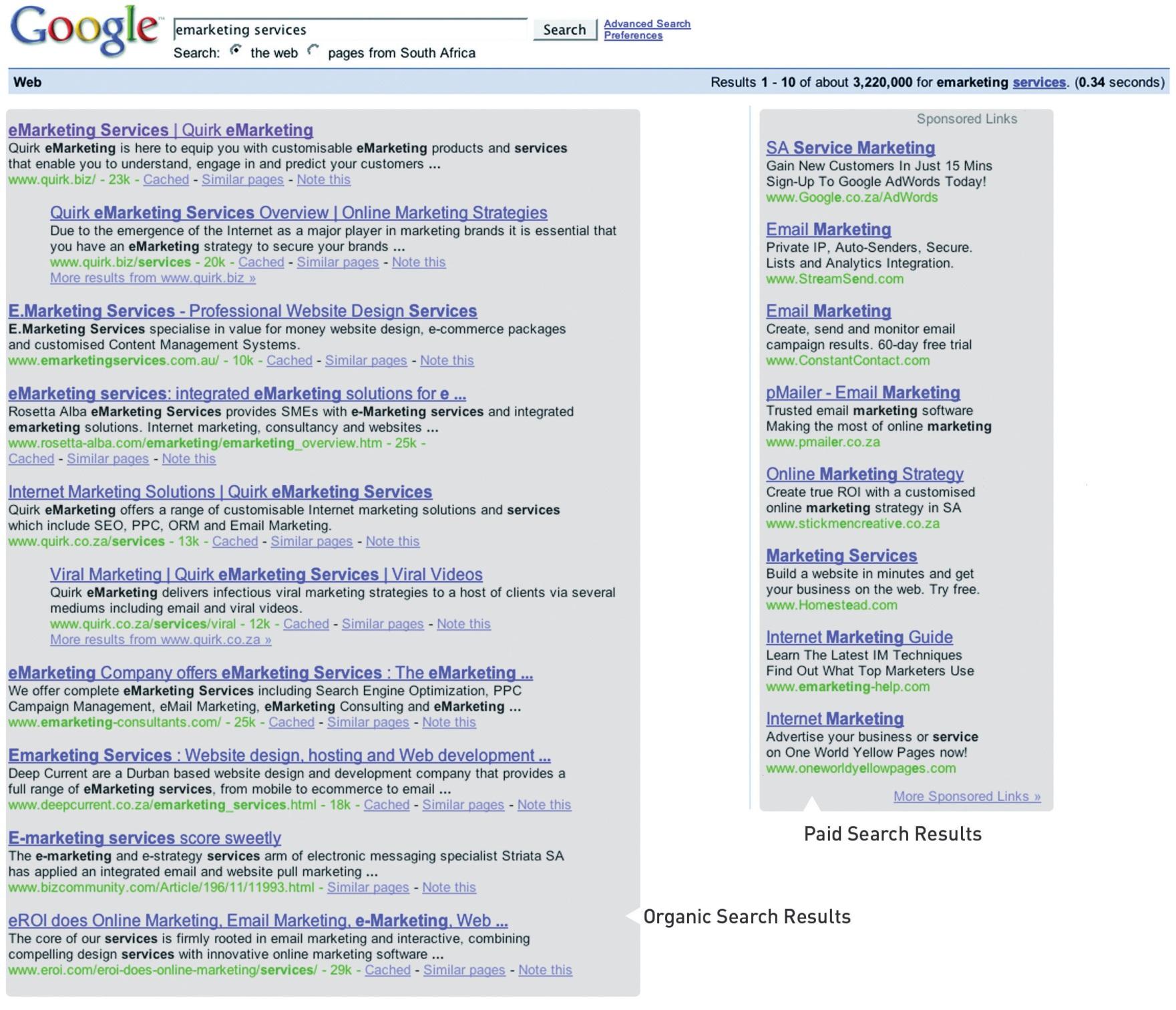A screenshot displays an old version of Google's organic search results for the query "e-marketing services." The vintage interface is characterized by a distinct font style and a grey backdrop for the search bar. The search has returned approximately 3,220,000 results in just 0.34 seconds. The results are ranked from 1 to 10 on the results page. Notably, the top search result appears in a purple, underlined font, suggesting that the user has previously visited this link. The URLs of the search results are displayed in green font. To the right of the organic search results, a sidebar includes several paid advertisements related to internet marketing services and guides. These details collectively highlight the distinctive aspects of Google's older search interface.